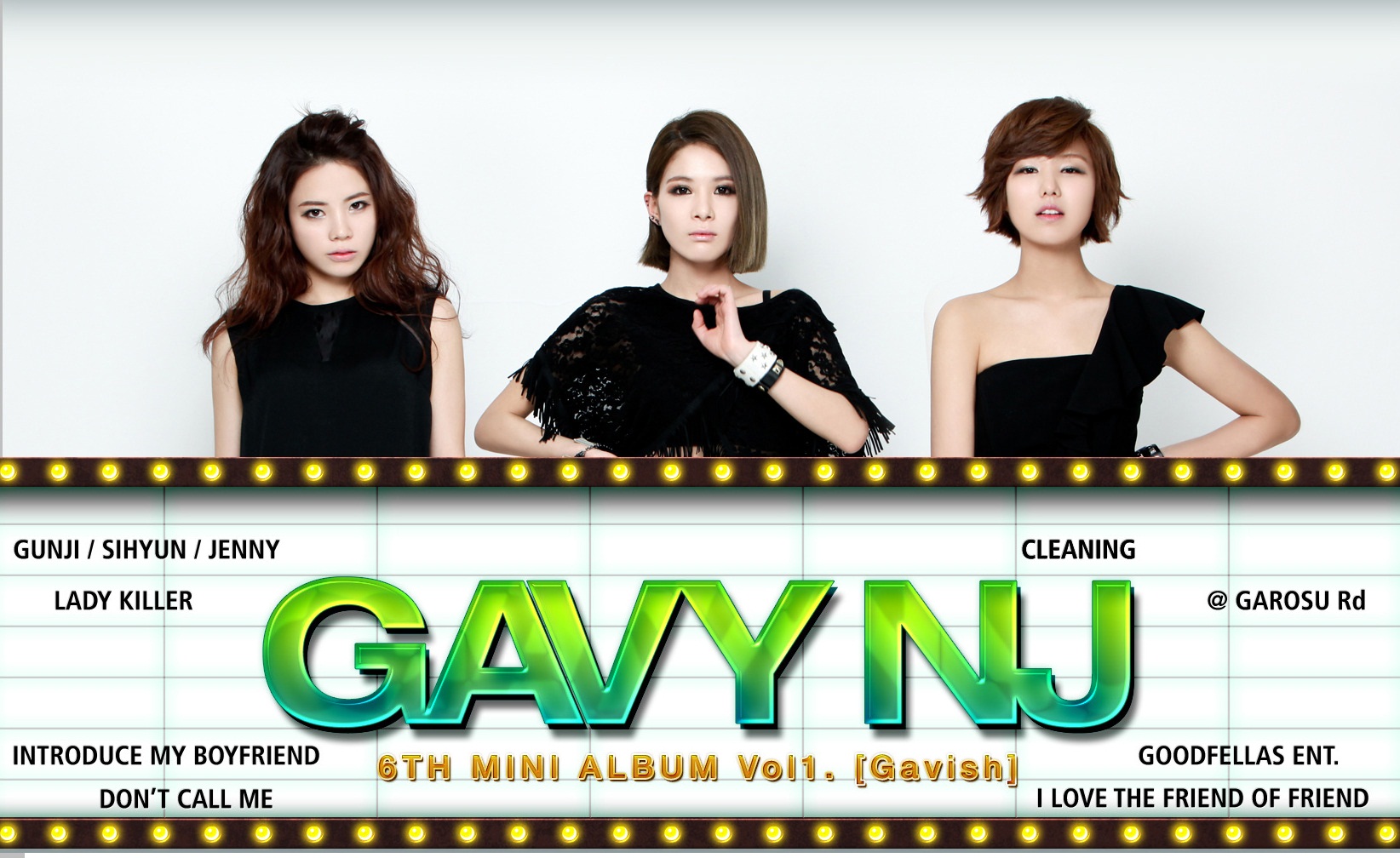This digital screenshot features a promotional poster for the girl group Gabby NJ, showcasing three Asian women standing next to each other against a white background. The women are dressed in black outfits with varying styles and lengths. The woman on the left dons a black sleeveless dress and has the longest hair. The middle woman sports a shawl-like neck dress with fringes that expose her elbows, and has medium-length hair. The rightmost woman wears a short-sleeved black dress over her left arm and has the shortest hair of the trio.

The text in the image includes the group's name "Gabby NJ," prominently displayed in large green and light green letters near the bottom. Additional text lists song titles such as "Lady Killer," "Introduce My Boyfriend," "Don't Call Me," "I Love Friend of Friend," and "Cleaning." It also notes that this is their 6th mini album, titled "Gavish." The names Gunji, Siyoon, and Jennie appear on the left side, which are presumably the names of the members. The poster suggests they are managed by Good Fellas Entertainment.